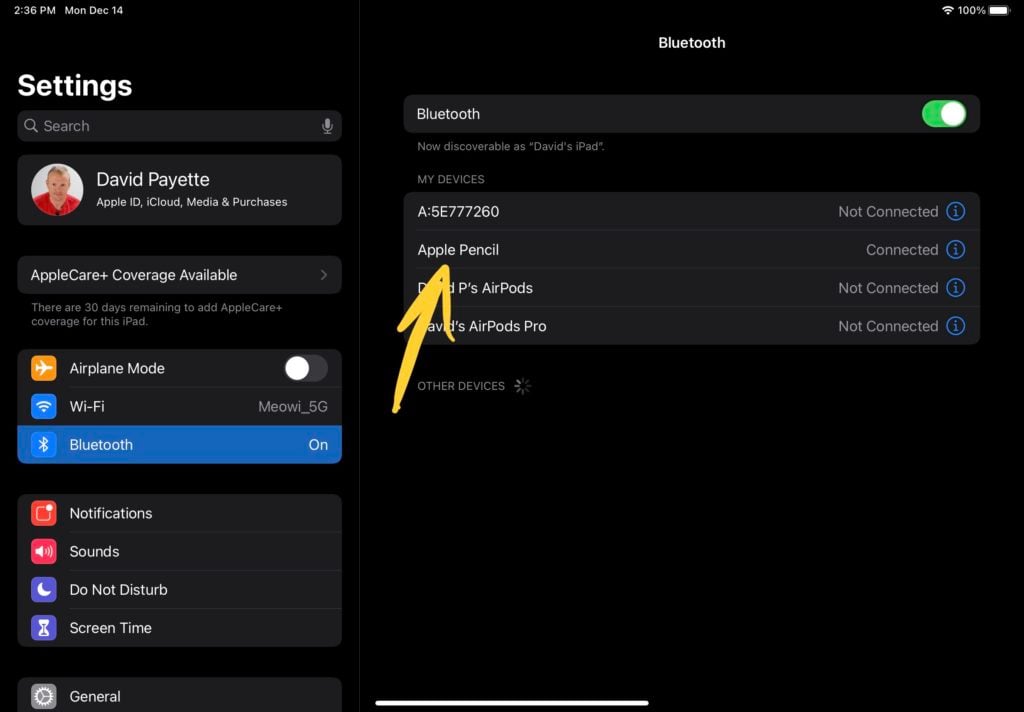This image is a composite screenshot capturing a settings page, seemingly from an Apple device. On the left side, the interface displays a header titled "Settings" written in white. Directly beneath the header, there is a dark grey search bar for quick access to settings options. Below the search bar, the Apple ID section is prominently displayed, featuring a circular profile picture of a white man identified as David Payette. Accompanying the profile picture, the text reads "Apple ID, iCloud, iTunes & App Store."

Below this section, there is a grey notification bar that states "AppleCare+ Coverage Available," suggesting an advertisement or a reminder for the user to subscribe to AppleCare+. 

Further down, the screenshot lists various settings options organized into sections. The first section includes essentials such as "Airplane Mode," "Wi-Fi," and "Bluetooth." Following that, another section encompasses general functionalities labeled "Notifications," "Sounds & Haptics," "Do Not Disturb," and "Screen Time."